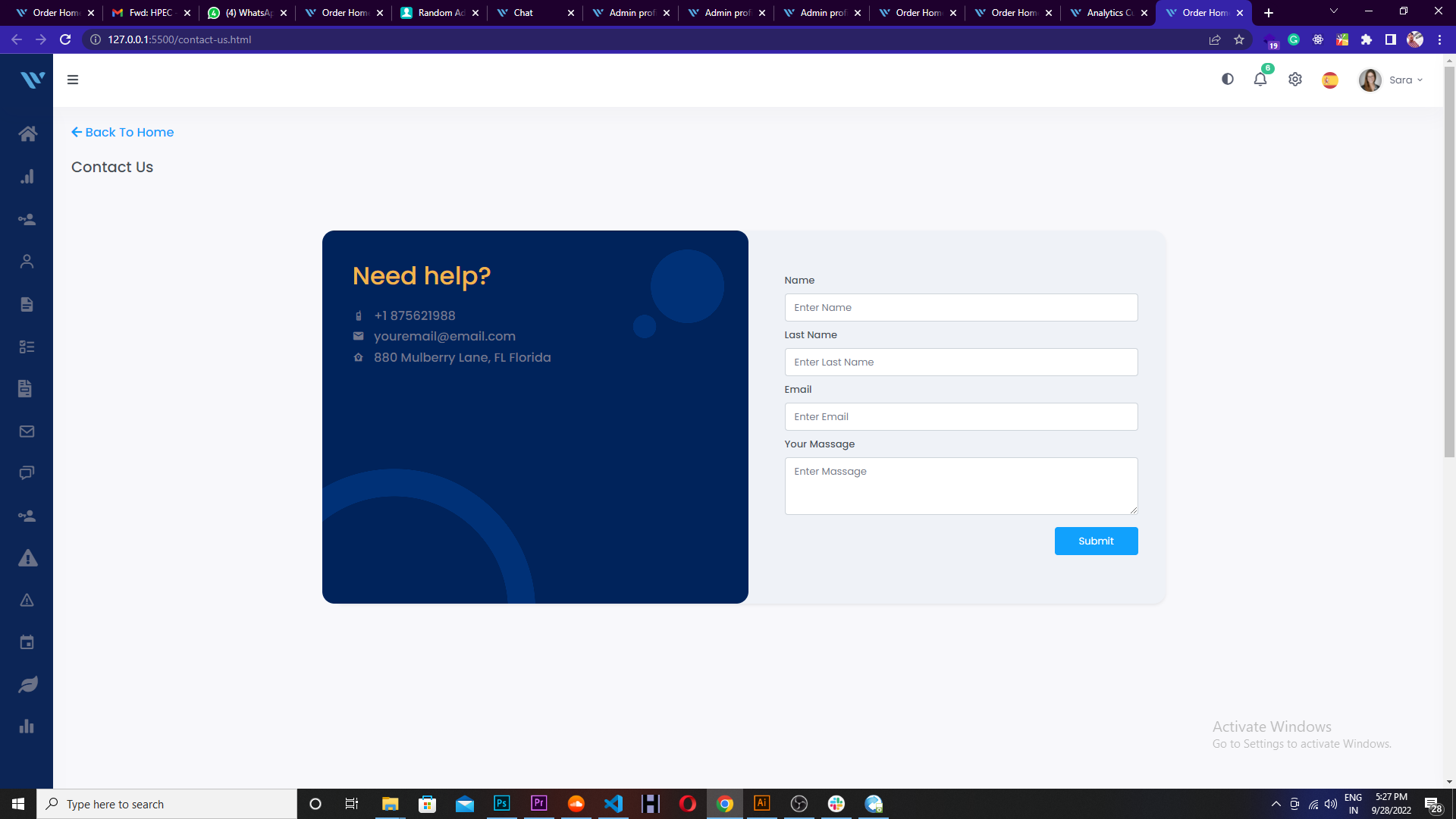This screenshot captures a computer screen displaying a webpage titled "Contact Us." The URL in the address bar reads "contact.us.html," indicating that the user is viewing an HTML file. 

At the top left corner of the webpage, there is a menu drop-down icon depicted by three horizontal lines. Directly below this, there's a blue "Back to Home" text accompanied by a leftward pointing arrow. Further down, in bold black text, the headline "Contact Us" is prominently displayed. 

The user's browser shows an abundance of open tabs, at least 10 are visible, with the currently selected tab labeled "Order Home."

The main content area of the page features a dark blue box with light blue circle accents. Inside this box, in vibrant orange text, it reads "Need Help?" Below this message, there's a contact phone number "+1 875 621 9988" in gray text, along with a small phone icon to its left. Further down, a mail icon is situated next to the placeholder email address "your.email@email.com." At the bottom of this section, a home icon is displayed next to the address "880 Mulberry Lane, Florida."

To the right of the blue box, there are several input fields designed for visitor interaction. These fields are labeled for the user's first name, last name, email, and message, followed by a submission button to send the entered information.